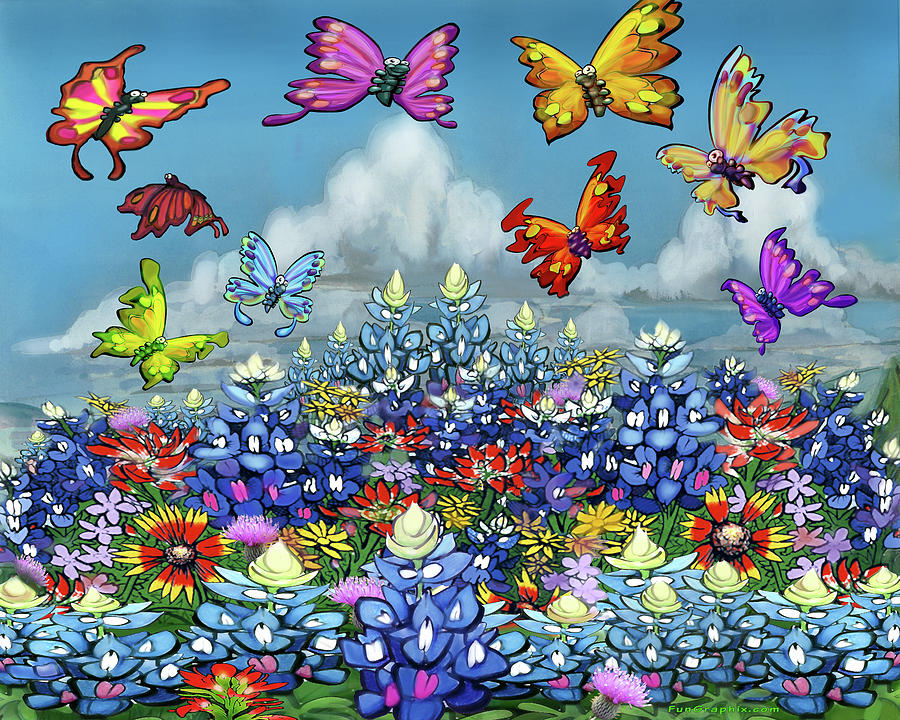This vividly colorful, stylized illustration, likely computer-generated, captures a fantastical garden scene brimming with life. A dense, vibrant field of wildflowers in blues, purples, yellows, pinks, and reds stretches across the bottom, showcasing a variety of petal shapes and plant structures. Above, ten uniquely colored butterflies with cartoonish white eyes and black pupils flutter gracefully. Their wings display a spectrum of hues, including green, blue, deep red, reddish with yellow stripes, purple with a blue body, yellowy brown, bright yellow with blue accents, and lilac with purple dots. The backdrop is a bright blue sky adorned with fluffy, white anvil-bottomed cumulus clouds, enhancing the whimsical and richly detailed atmosphere of this watercolor-styled poster.